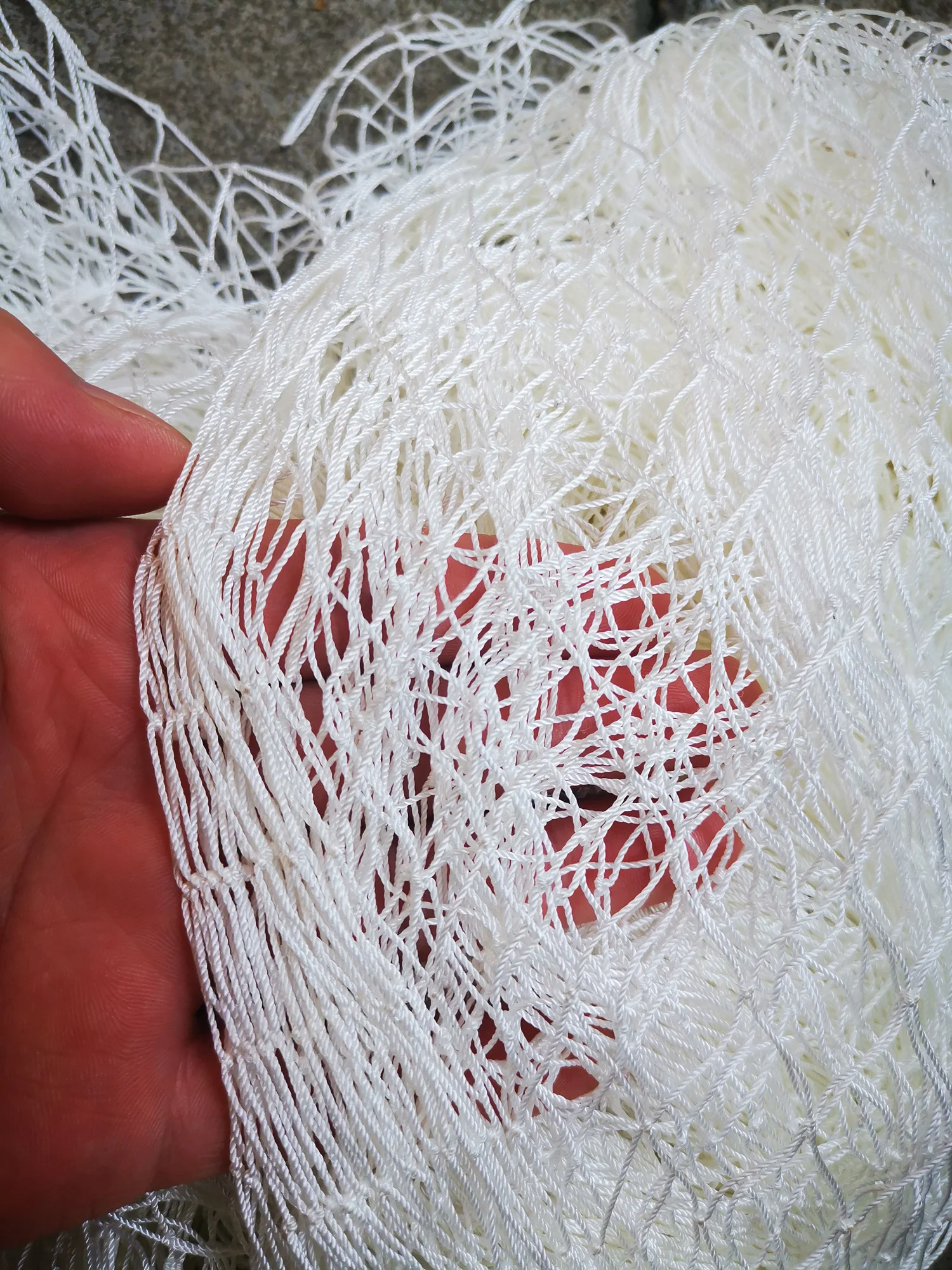This close-up, overhead image vividly showcases a brown hand with short fingernails holding a tangled mass of fine, white mesh that evokes the texture of a volleyball net. The mesh, made of very thin nylon strings, is tangled and piled chaotically, enveloping the fingers. The hand, predominantly visible on the left side of the frame, reveals a partial view of the palm and a side glimpse of the thumb. The translucent quality of the mesh allows the reddish-pink tones of the hand to subtly show through. Surrounding the hand and mesh, the background includes hints of a tightly woven gray carpet with possible speckles, adding texture to the otherwise blank space around the netting.